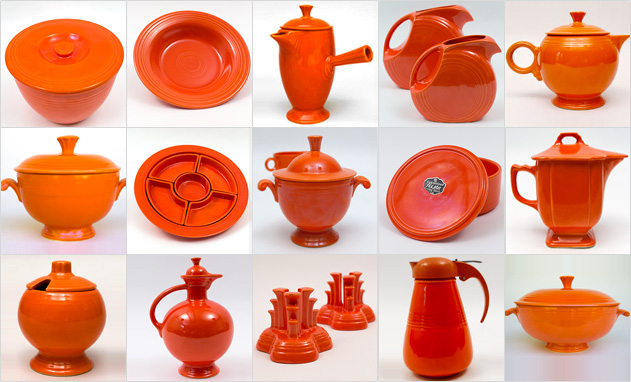This image is a collage of 15 individual square images, each set against a white background, showcasing a collection of orange to red kitchenware. The kitchen items vary in shades from deep orange to red and include an array of ceramic-looking and possibly plastic pieces. These items appear to be from the same brand as indicated by a partially visible label on one of the lids, though the brand name is unreadable. Key items include a red bowl with a lid, a deep dish, a tea kettle with a long handle, and several pitchers of varied shapes including a turtle shell-shaped pitcher. There's also a round tea kettle with a curved handle, a soup pot, a compartmentalized plate with five sections, and multiple serving dishes and pots with lids. Some pieces are open like plates and bowls, while around 45% of them have matching lids. The collection also features two red stands and various pitchers prominently designed for pouring liquids. The consistent orange-red color palette ties the eclectic assortment of kitchenware together, despite minor variations in hue.